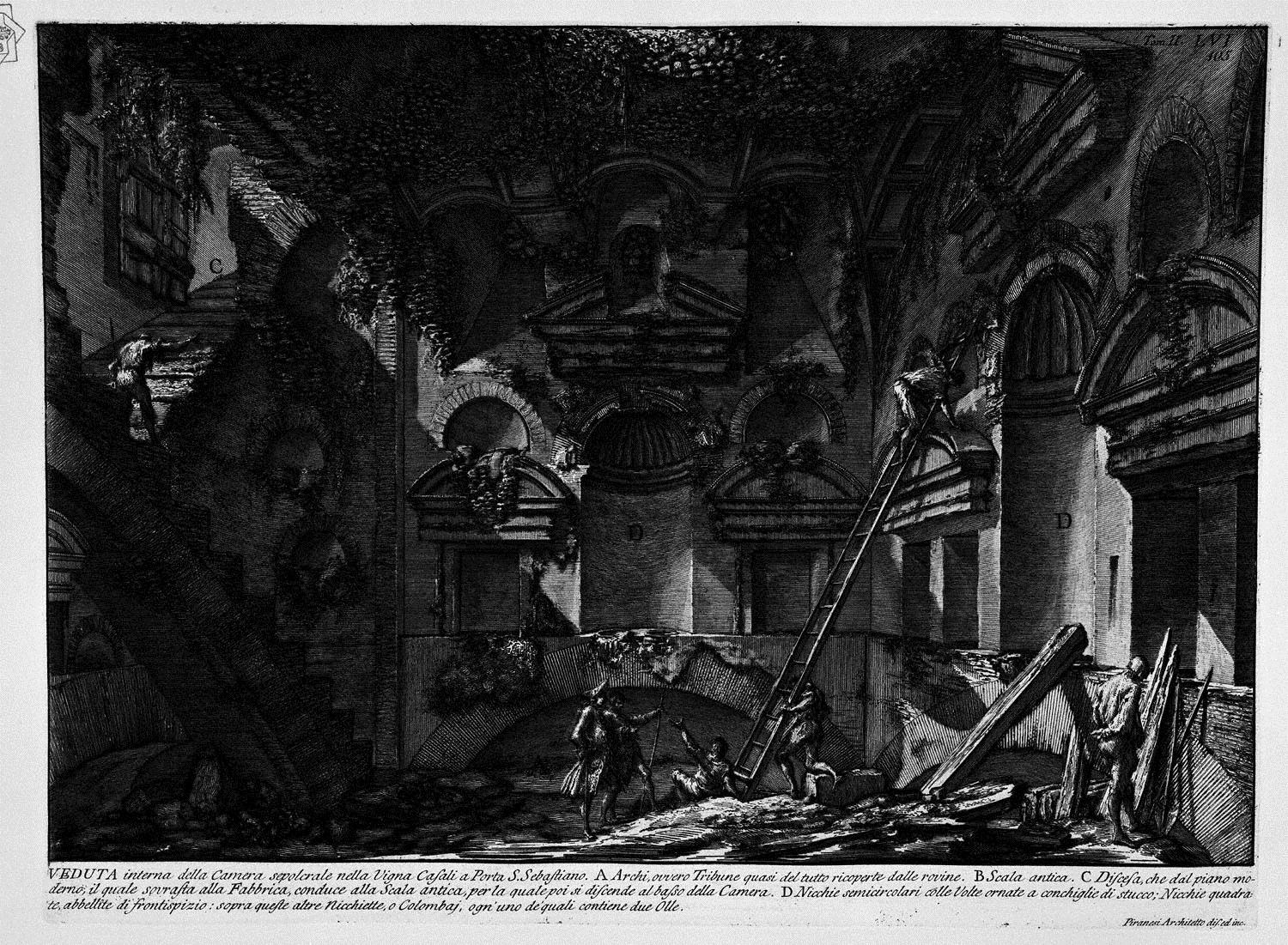The image is a detailed, monochromatic artwork, likely a black-and-white sketch or woodcut, depicting the interior of a gothic or medieval building. The room is dimly lit, with shafts of light penetrating through unseen windows, casting intricate patterns on the high, curved ceilings and arches. Central to the image is a ladder extending diagonally up to a wall, with a man perched at the top. Surrounding him, several other figures stand amidst debris and lumber, gesturing and possibly working on the building's renovation or repair. The scene has a gloomy, claustrophobic atmosphere, compounded by the heavy use of greys and blacks. At the bottom of the image, there is a block of text, possibly in Italian, which includes the phrase "Veduta interna della Camara," indicating it is an internal view of the room. The text consists of around three lines, adding context or a title to the scene.